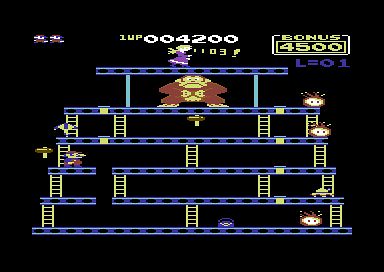This image appears to be a screenshot from an older video game, characterized by its retro, pixelated art style. At the center of the action is a small character reminiscent of Mario, navigating a series of six tiered platforms connected by ladders. Each platform teems with different monsters that challenge the character's progress as they ascend. Below the top platform, a formidable monkey, resembling Donkey Kong, stands guard. Crowning the scene at the apex is a princess, presumably the character that must be saved, highlighting the primary objective of the game.